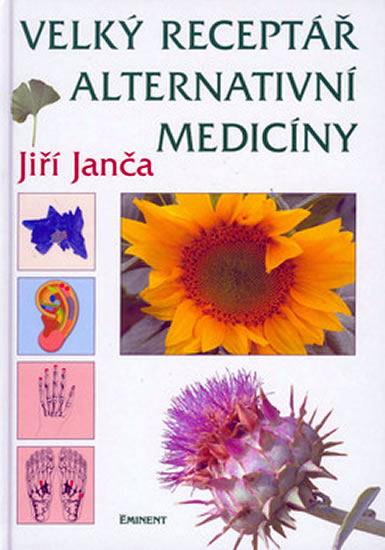The book cover features the title "Velki Receptar Alternativni Medicini" in dark green font, presented in a non-English language and indicating a focus on alternative medicine. The author's name, "Giri Janka," is printed underneath the title in red font, with a green leaf overlaying the first letter. The cover, set against a white background, includes several distinct images: on the left side, there are four vertically aligned squares. The top square displays a bluish geometric structure; the second features a rainbow-colored ear diagram with a light blue background and multicolored dots; the third shows a skeletal hand with pink fingernails; and the fourth contains a skeletal foot with red dots. To the right of these squares is a large rectangular image of a bright yellow sunflower, and beneath it is a spiky flower that is purple and red. At the bottom in tiny green font, the publisher's name, "Eminent," is printed.